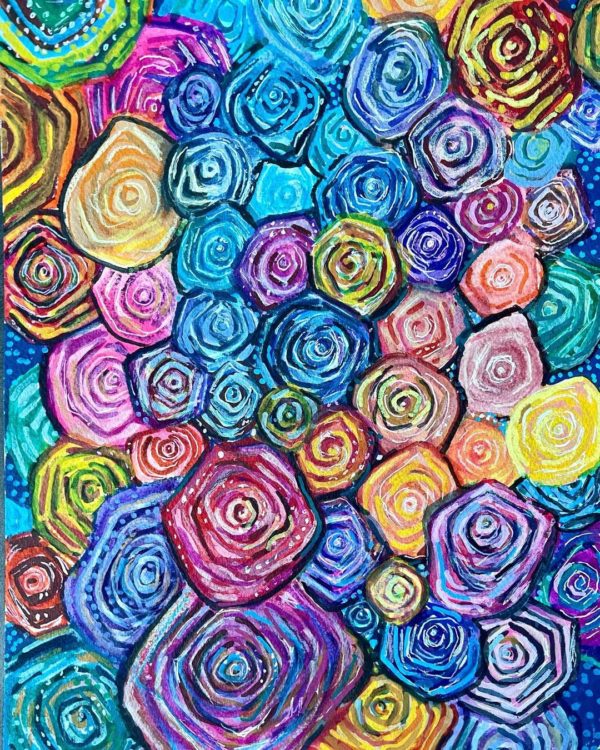This vibrant painting, possibly created with oil or mixed mediums, features an array of abstract flowers with vividly colored, concentric circular shapes representing petals. The flowers cover the entire canvas in a tightly packed formation, extending off the edges, and are rendered in an array of colors including purple, blue, yellow, pink, teal, green, and red, with some showing hints of burgundy, gold, and brown. Each flower swirls inward, creating an illusion of depth with darker black areas and lighter accents of white. Despite the rough and amateur style, characterized by rough shapes and dotted details, the composition is rich and colorful, filling the canvas with around 40 to 50 roses of various sizes. The very few visible parts of the background reveal dark blue hues with light blue highlights, adding further depth to the artwork.